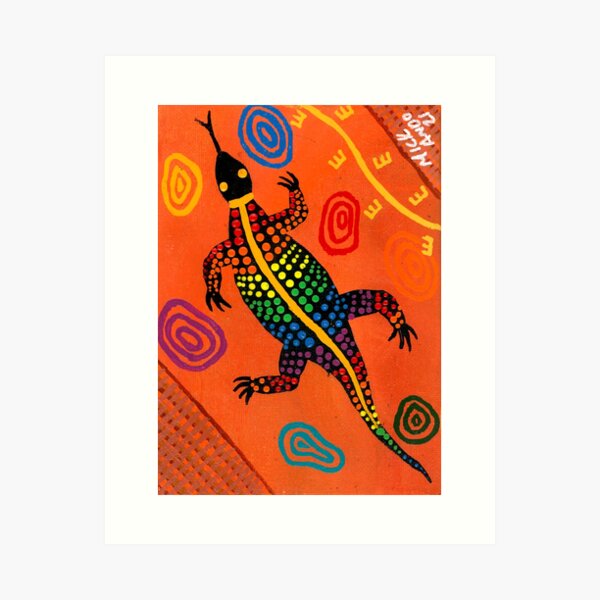This image features a vividly detailed piece of artwork by indigenous artist Mick Ando, signed in the upper right corner with "Mick Ando '21," although the signature appears upside down. The central focus is a stylized gecko adorned with a striking array of rainbow-colored polka dots in red, orange, yellow, green, blue, and purple, repeating in sequence. The gecko has a black head and tongue, black feet, yellow eyes, and is marked by a yellow horizontal band across its neck that extends into a vertical yellow stripe running down the length of its body. Spiraling around the gecko are six circles in vibrant shades of blue, yellow, purple, red, teal, and black. The background is a bold orange, providing a stark contrast to the multicolored elements. Additionally, a curved yellow wavy line, paralleled by backwards capital "E" motifs, intersects at the top right corner of the artwork. The lower left corner features a detail of what looks like a woven basket in white, off-white, and red, with red lines and dots extending from this corner, enriching the texture of the overall composition.